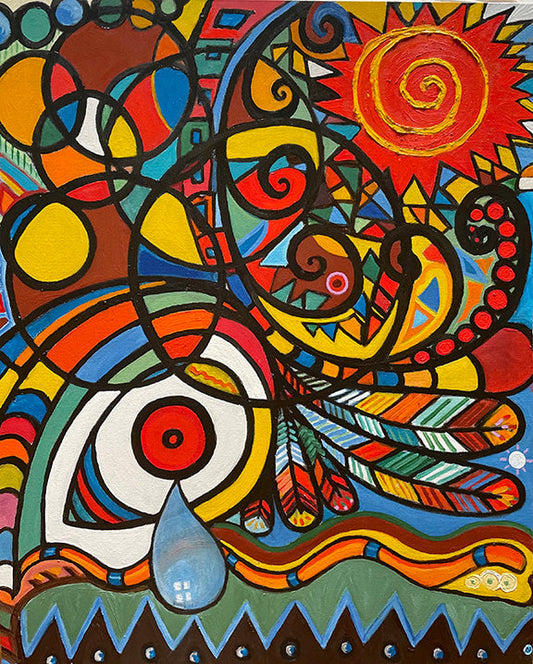This oil painting bursts with bright, primary colors and intricate, abstract details. Dominated by motifs such as feathers, paisley patterns, starbursts, and numerous concentric circles, the image evokes a stained-glass effect through its geometric shading within larger shapes. The color palette prominently features vivid mint green, baby blue, orange, yellow, alongside bold black outlines, and touches of brown and white.

In the upper right corner, a striking multi-spiked orange sun with a yellow spiral centerpiece commands attention. The lower left, in contrast, showcases a large, stylized eye with a blue teardrop, surrounded by peacock-like elements: feathers in hues of blue, red, green, yellow, purple, brown, and black, mimicking the eye patterns found on peacock wings.

A notable feature is the orange snake with blue bands, slithering horizontally above what appears to be a wavy green mountain ridge at the bottom, adding an earthy, mystical layer to the composition. Further details include black mountains topped with blue accents and central blue dots, suggesting a Native American influence. Overall, the piece is a vibrant tapestry of colors and shapes, blending abstract beauty with deep, symbolic elements.